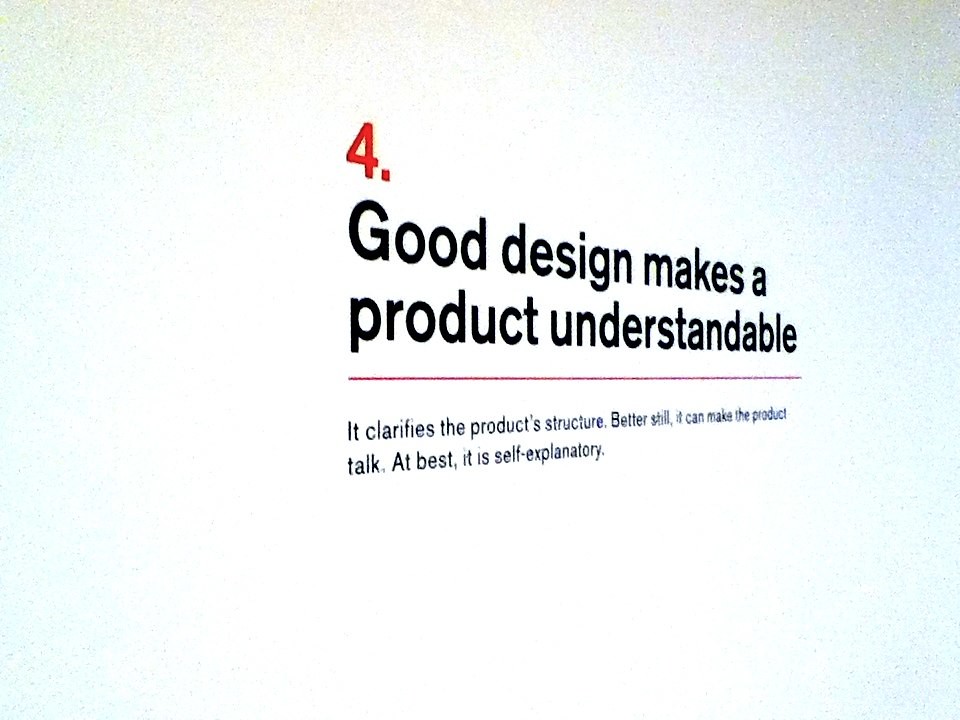The image depicts a presentation slide with a clean, white background, captured at an angle where the left side appears larger than the right. At the top of the slide, a red number "4" followed by a period is prominently displayed. Below this, two lines of black text read: "Good design makes a product understandable." A thin red line runs horizontally, visually separating the previous text from another two lines below. The bottom portion of the slide contains additional black text stating: "It clarifies the product structure, better still it can make the product talk, at best it is self-explanatory." The simplicity of the slide, combined with the clear separation of ideas using text and a red line, underscores the message about the importance of good design.